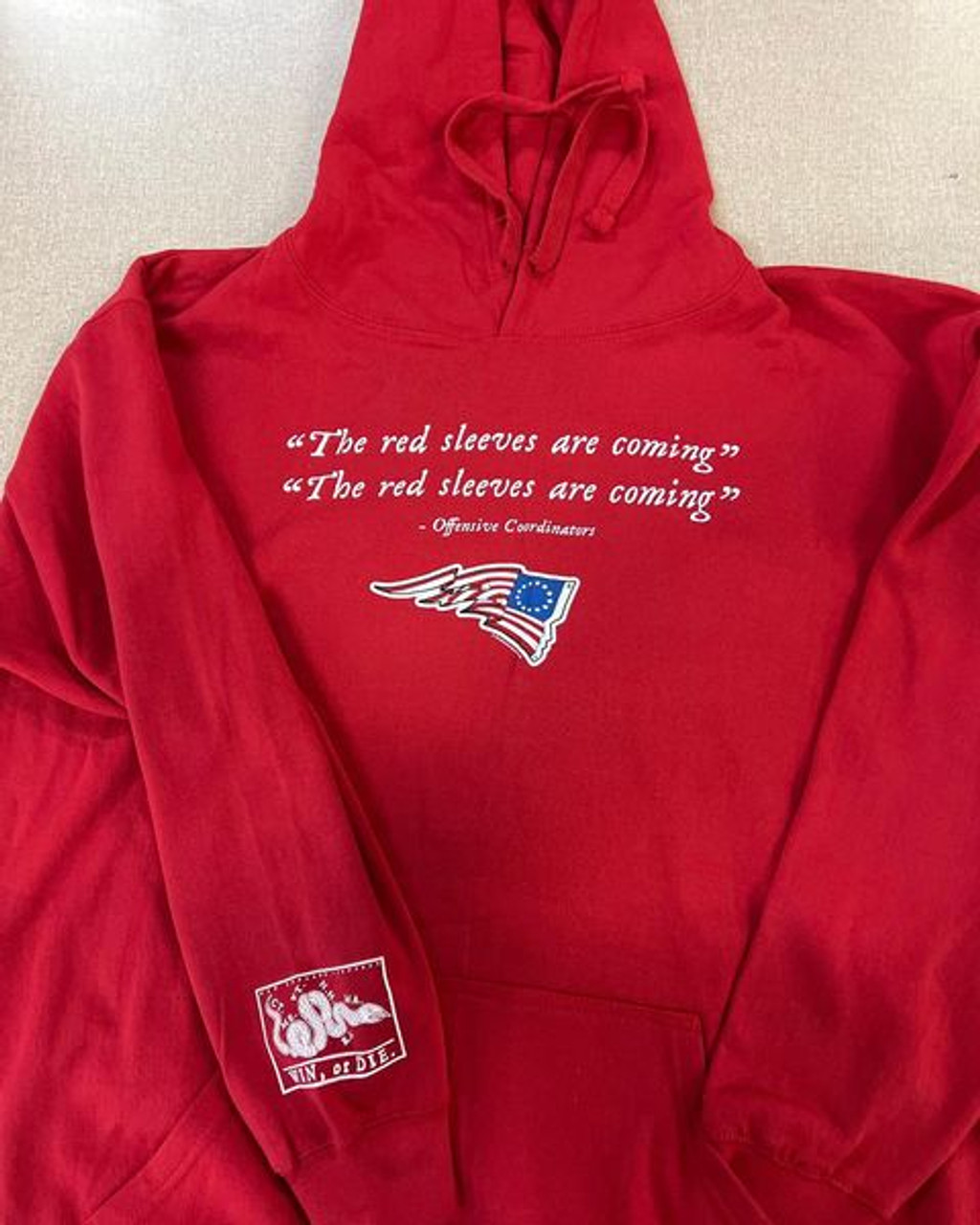The image features a bright red New England Patriots sweatshirt or hoodie, folded with the arms positioned forward, lying on a light gray-tan background, possibly a table or carpet. The sweatshirt prominently displays in bold white letters across the chest: "The red sleeves are coming," repeated twice. Below this phrase, centered in smaller text, it reads "Offensive Coordinators." Underneath this text, the design includes an image of the American Revolutionary flag with a stylized 13-star circle on a blue field, appearing ruffled as if waving. On the right sleeve near the cuff, there is an additional logo featuring a white rectangular patch with a coiled snake and the words "Win, or Die," underlined, a nod to historical symbols of resilience and defiance. The hoodie also has drawstrings near the top, completing its casual and patriotic design.